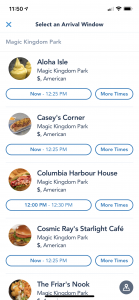The image is a slightly blurry screenshot of a smartphone displaying a dining reservation app for Magic Kingdom Park. At the top of the screen, the status bar shows the current time, Wi-Fi signal strength, and battery level. Below the status bar, text indicates a selection of arrival windows for various dining options.

Starting from the top, the first listing shows a reservation for 'Aloha Isle' with an icon of what appears to be a creamy dessert. The reservation is for 12:25 PM with additional times available. The next listing is for 'Casey's Corner,' featuring an icon of a sandwich, also available for reservations at 12:25 PM with more times listed. A third option, 'Columbia Harbour House,' is indicated with another sandwich icon and shows an available reservation window from 12:00 PM to 12:30 PM, along with more times. Another entry reads 'Cosmic Ray's Starlight Café,' marked with a hamburger icon and a reservation time of 12:25 PM, again with additional times available.

The final listing, partially cut off, is for 'The Friar’s Nook,' and appears to display an assortment of food items. All listed times are highlighted within blue circles, and the background of the app is white.